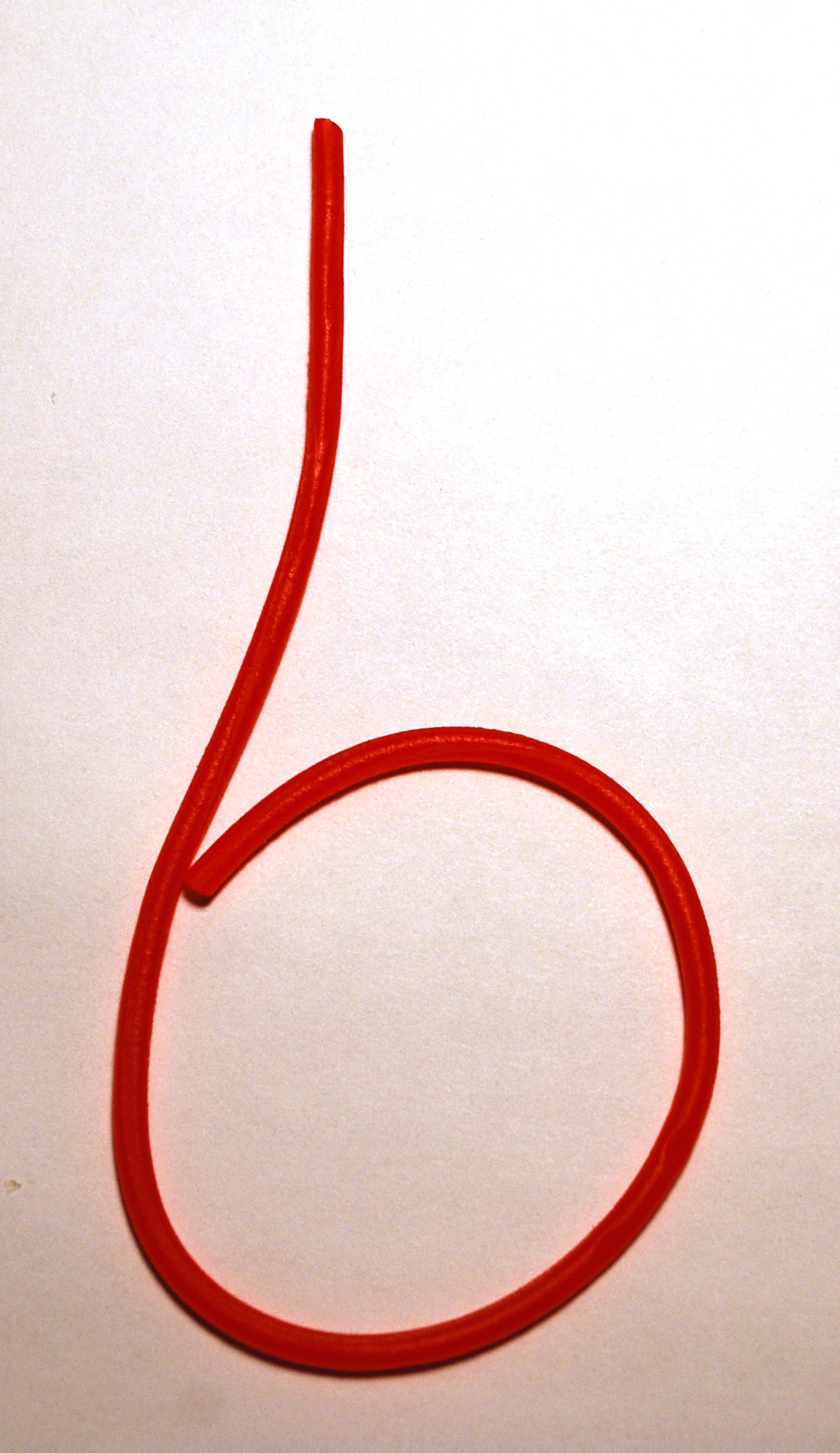This is a photograph featuring a dark scarlet, red tubing that forms the shape of the number six. The tube, which appears to be a piece of licorice or possibly a narrow, inconsistent hose, lies on a background that gradiates from a light off-white at the top to a darker, almost pinkish hue towards the bottom. The tubing starts from the top middle of the image, descends nearly to the bottom, and then loops back up to form a nearly perfect circle characteristic of the number six. The surface it's resting on is predominantly light grayish-brown, and while the exact material of the tubing is unclear, its inconsistent diameter suggests it might be something flexible rather than a solid tube. The top of the photograph appears brighter, gradually becoming darker towards the bottom, enhancing the prominence of the vibrant red tubing.